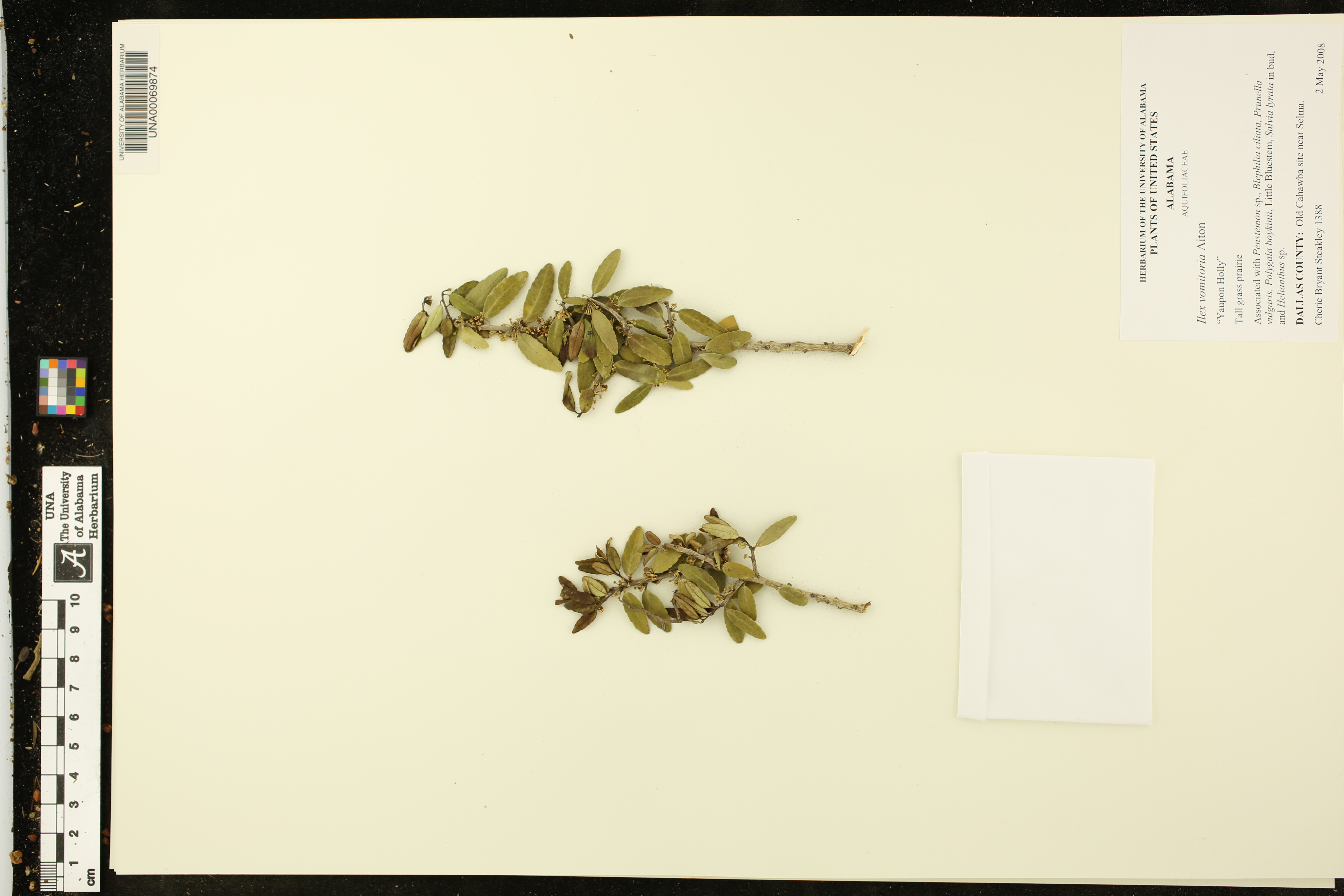This image is a detailed photograph of a catalog sample of greenery, possibly mistletoe or similar plants, from the University of Alabama Herbarium. The photograph features two green plant specimens displayed on a yellow paper background, with one plant larger than the other. There is a white folded pouch attached under the plants, possibly containing seeds. The image includes a barcode in the top left corner and a detailed chart in the top left showing a scale from 0 to 10 centimeters. The background is black with a multi-color rainbow design on the left side. The text on the image, which is small and horizontally oriented, reads “Plants of the United States, Alabama, Dallas County, chat bus site near Selum. Sherry Bryant Steeke, 1388. 2 May, 2008,” and also mentions “Herbarium of the University of Alabama” along with some additional Latin terminology.